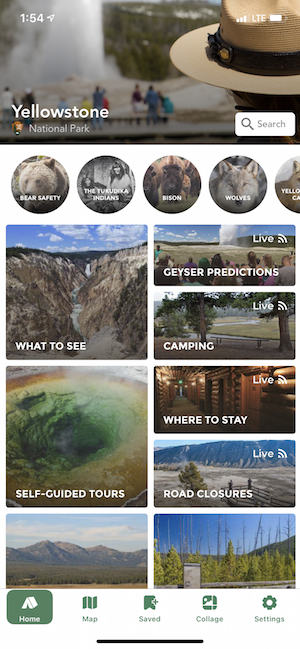The image depicts a website banner showcasing an outdoor scene. The top section features a scenic backdrop with a person in the foreground, seen from behind, wearing a straw hat with a black band. This individual is gazing out over what appears to be a waterfall surrounded by numerous people. The banner displays a timestamp of 1:54, an LTE signal indicator, and a battery icon. 

Prominently, the banner reads "Yellowstone National Park," with a search feature consisting of a small white rectangle with a magnifying glass icon and the word "search" in gray print. Below the banner, there are three circular icons with various images and captions: one reads "Bear Safety," another "Kodaka Indians" with a bison illustration, and another labeled "Wolves." A partially visible fourth circle displays "Yellow" with "C8" underneath.

Further down, there's a section titled "What to See," featuring a picturesque landscape with mountains, sky, and a river. At the bottom of the image, there are more options labeled "Self-Guided Tours," "Geyser Predictions," "Camping," "Where to Stay," and "Road Closures," each accompanied by relevant icons or images. The navigation menu at the bottom includes options for "Home," "Map," "Saved," "Collage," and "Settings."